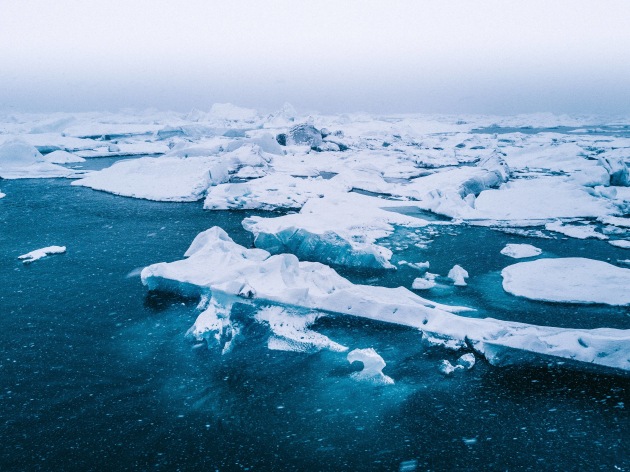An aerial view captures a frigid seascape likely in Antarctica or a similar polar region, characterized by a striking contrast of elements in a wintery scene. The vast ocean, a mesmerizing aquamarine blue, hosts numerous large, broken chunks of ice floating freely, with some massive icebergs partially submerged, revealing their impressive size under the surface. The sky above transitions from a grayish-white at the top to a deeper blue lower down, adding to the cold atmosphere. Distant snow-capped mountains provide a dramatic backdrop, their white peaks standing out against the sky. The landscape includes scattered glaciers and smaller ice caps, with no central landmass, just a network of ice and water. The scene lacks any visible wildlife, adding to the stark, serene beauty of this frozen wilderness.